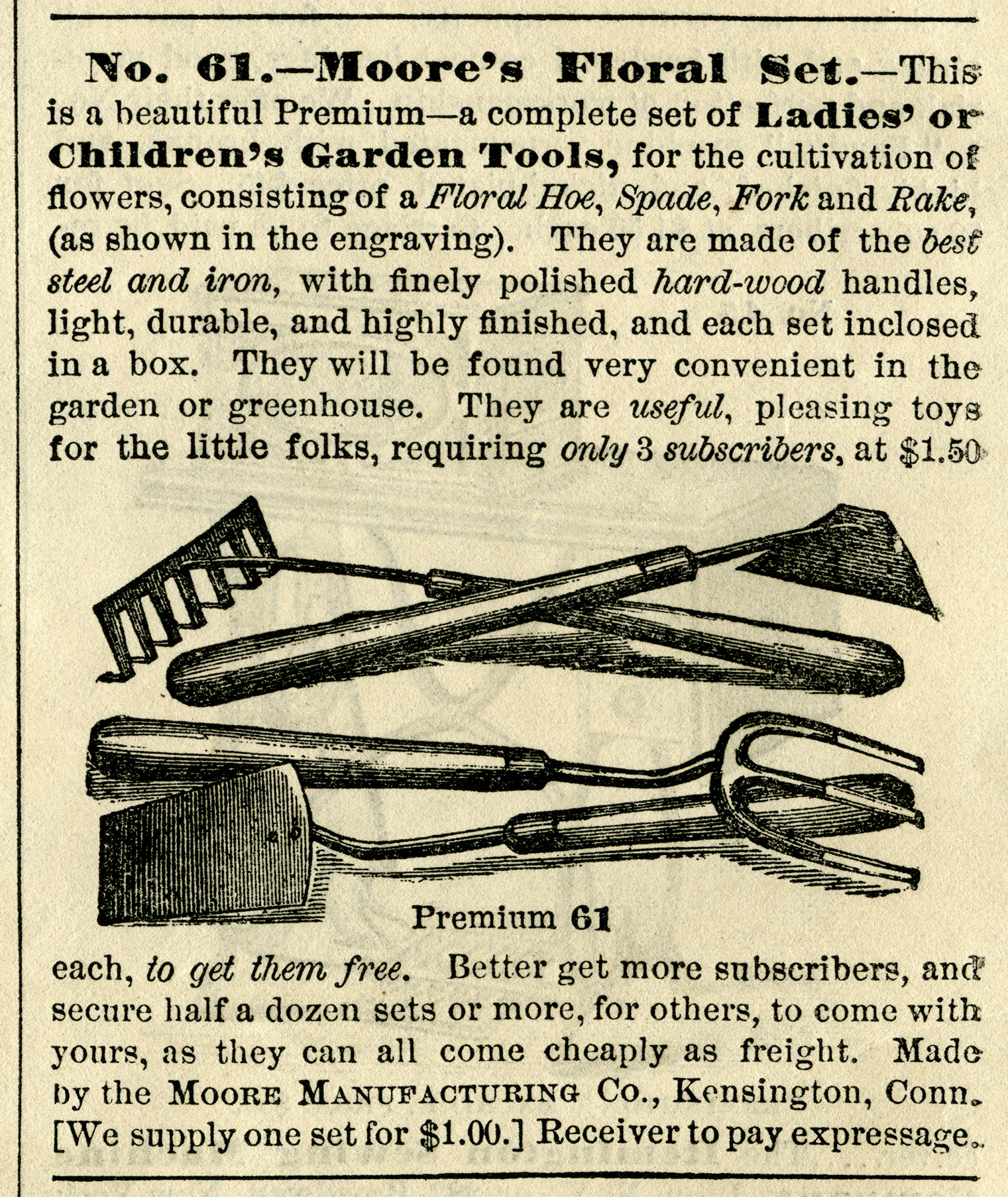The image depicts an old, yellowed newspaper clipping, most likely from the 1800s, showcasing an advertisement for "Number 61 Moore's Floral Set." The advertisement highlights a beautifully crafted premium floral tool set designed for ladies or children to cultivate flowers. The set includes a floral hoe, spade, fork, and rake, each made from high-quality steel and iron with finely polished hardwood handles that are light, durable, and highly finished. These tools are illustrated in the ad with detailed engravings. Described as useful and pleasing toys for children, the set is marketed with an offer: acquiring three subscribers at $1.50 each allows one to receive the set for free, with additional sets available at a minimal cost. The advertisement notes that the tools would be convenient for use in gardens or greenhouses and mentions the Moore Manufacturing Company based in Kensington, Connecticut. The ad also includes specific details on pricing and express postage.